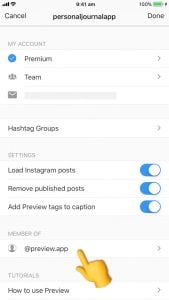The image is a screenshot taken on a mobile phone, with the battery status at 100%. At the top of the screen, there's a header featuring three elements: "Cancel" on the left, "Personal Journal App" in the center, and "Done" on the right. These are likely navigation links rather than buttons.

Beneath the header, the text "My Account" is displayed alongside a blue verified check mark labeled "Premium." There is a caret next to this text, suggesting that clicking it expands a menu with more options for premium features. 

Following this is the "Team" section, also accompanied by a caret for additional menu options. Below "Team," there is a gray icon that appears to represent an email inbox, but the email address is obscured by a gray box, making it unreadable.

Next, the "Hashtag Groups" section is listed with an expandable caret. This is followed by the "Settings" section, which contains several toggle options. Each toggle—"Load Instagram Posts," "Remove Published Posts," and "Add Preview Tags to Caption"—is highlighted in blue, indicating they are all turned on.

After "Settings," there is a "Member of" section that displays a profile avatar next to the text "preview.app." A finger icon points towards this text and there is a caret to the right, signifying that more options are accessible via another screen.

The subsequent section is titled "Tutorials," with a subheading "How to Use Preview" accompanied by another caret for further navigation options. The image cuts off at this point, leaving the rest of the content unseen.

Overall, the screenshot appears to be from the user interface of a mobile app designed for personal journaling, featuring various settings and account management options.